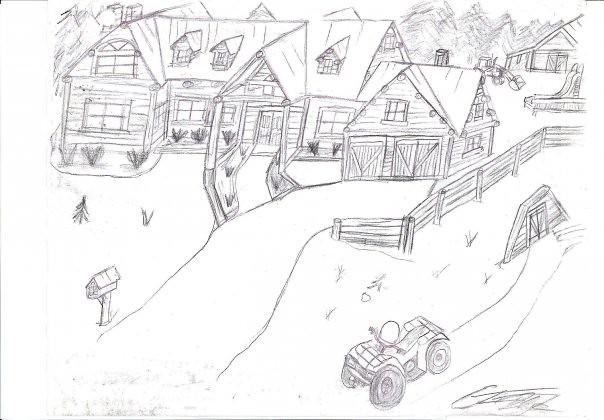The image depicts a detailed pencil sketch on a white background, likely fine paper or canvas, showcasing a large wooden log cabin or farmhouse. The architecture is characterized by angular, pointy roofs and multiple sections, including a single storey with attic windows embedded into the sloping roof. The house features several windows, a front walkway, and a long driveway leading to a mailbox shaped like a barn. The property includes additional structures, such as a barn area and a building with two wooden garage doors. Various elements outside the house contribute to a rural setting, including a ride-on lawnmower or ATV and a sliding board near the structures. There is an artist's signature on the bottom right, adding a personal touch to the artwork.